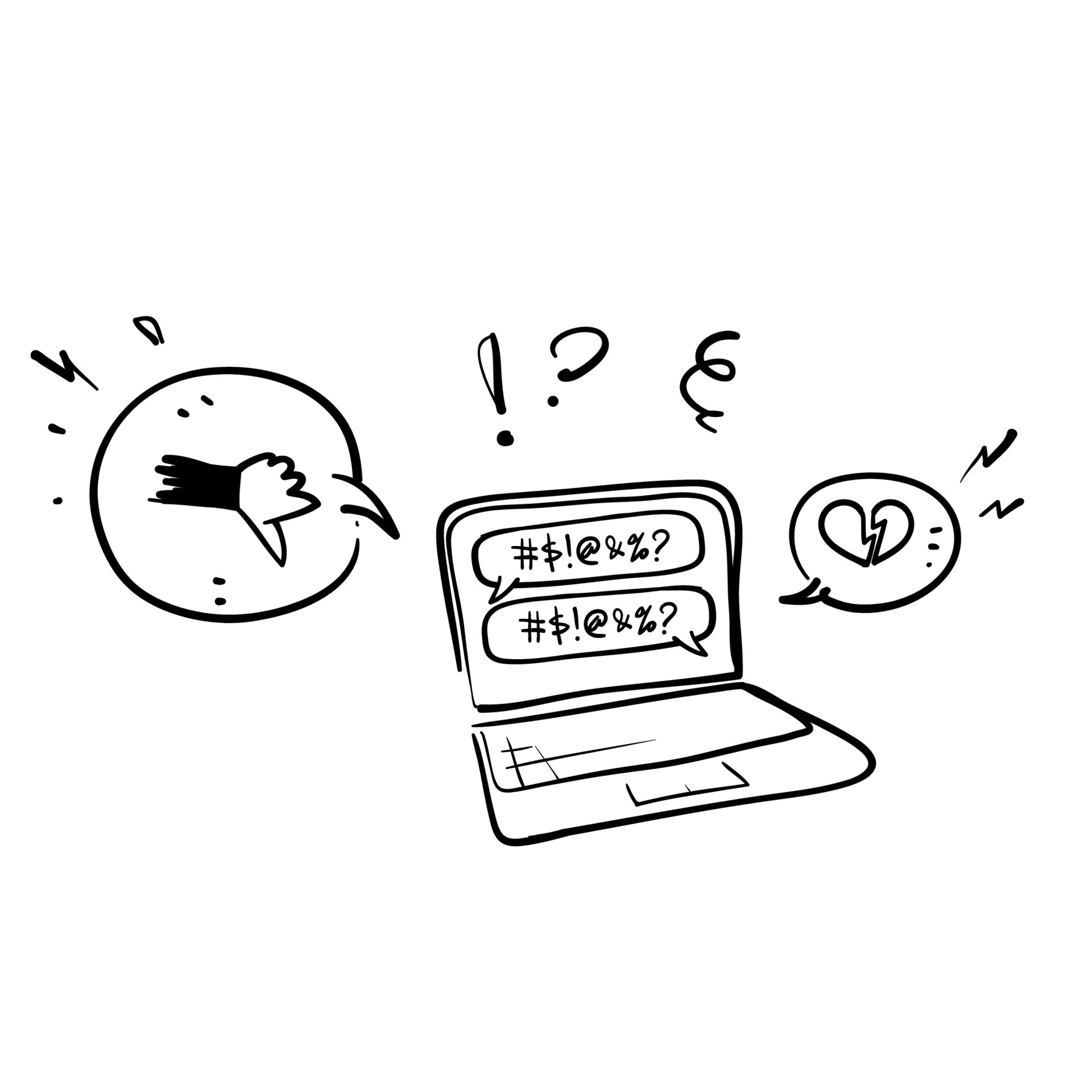This black-and-white drawing, which could be either computer-generated or hand-drawn, features a simplistic and somewhat whimsical depiction of an open laptop without a border or background coloring. The laptop's edges are slightly curved and irregular, adding to its quirky, non-lifelike appearance. On the screen, two identical speech bubbles filled with nonsensical symbols—# $ ! @ & % ?—appear, with one bubble emerging from the top left and the other from the bottom right. To the right of the laptop, another speech bubble contains a broken heart icon, accented by lightning bolts. On the left, a similar bubble showcases a thumbs-down sign, also accompanied by lightning bolts. Above the laptop, hover an exclamation point, a question mark, and a squiggly line, further emphasizing the chaotic and expressive nature of the drawing. The keyboard is only partially visible, with minimal detail, reinforcing the sketch's cursory and amateurish style.